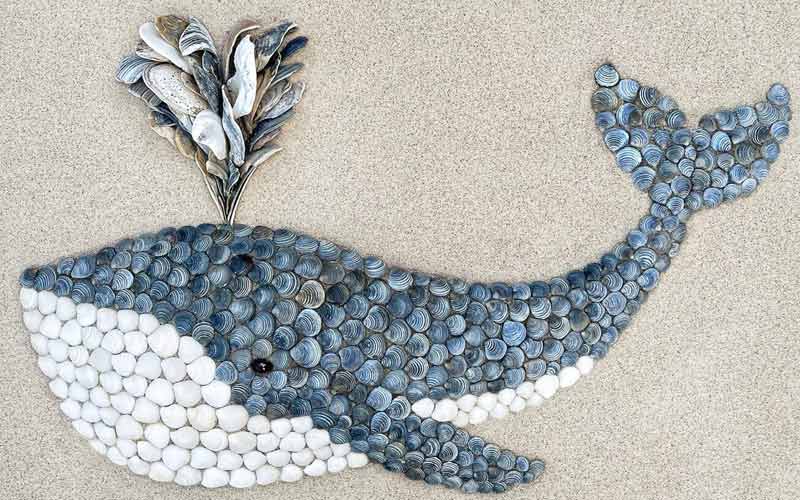This photograph captures a meticulously crafted sculpture of a blue whale created entirely from various seashells, set against a smooth sandy backdrop. The image is taken from a bird's-eye view, offering a clear, straight-down perspective of the artwork, which faces to the left. The whale's body is composed of blue and white shells arranged to mimic the creature's natural coloring. Blue oyster shells form the top half of the whale, while the underbelly is constructed from tightly packed white clamshells, giving it a textured, realistic appearance. A single black shell serves as the whale's eye. Adding to the whimsical nature of the piece, a jet of water emerges from the whale's blowhole, fashioned from an array of long, irregularly shaped shells in shades of white, brown, black, and gray, simulating the look of splashing water. The overall impression is of a charming, cartoonish marine figure rendered with great attention to detail and natural materials.